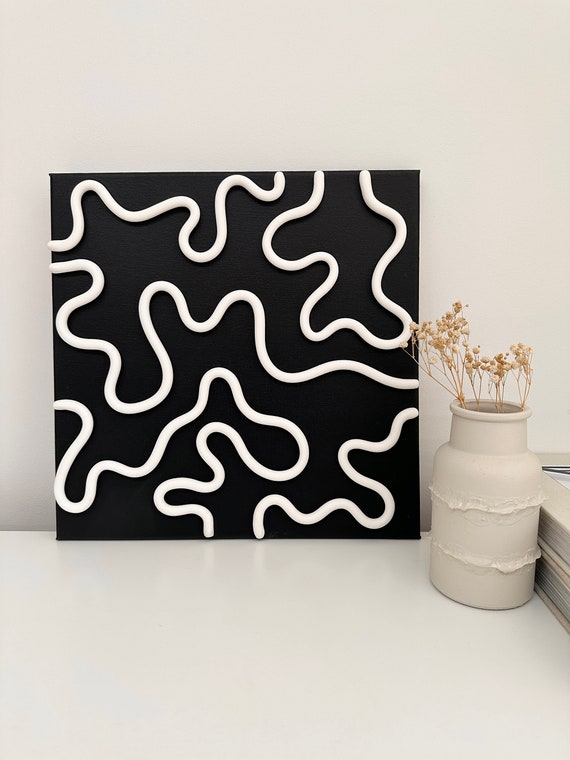This photograph captures a meticulously staged interior that resembles a design showcase or an art gallery. Dominating the composition is a square-shaped canvas with a solid black background featuring an intricate, non-intersecting network of white squiggly lines that appear almost three-dimensional. The canvas, leaning against a light grey wall, sits on a pristine white floor, adding contrast and depth to the scene. Adjacent to the artwork is an unusually tall, beige vase or old milk jug, adorned with two ridged lines and filled with dried, slightly wilted plants. This vase is positioned next to a matching beige ledge composed of several stacked wooden pieces, creating a textured, layered effect. The harmonious beige tones and artistic elements combine to form a visually engaging and thoughtfully curated space.